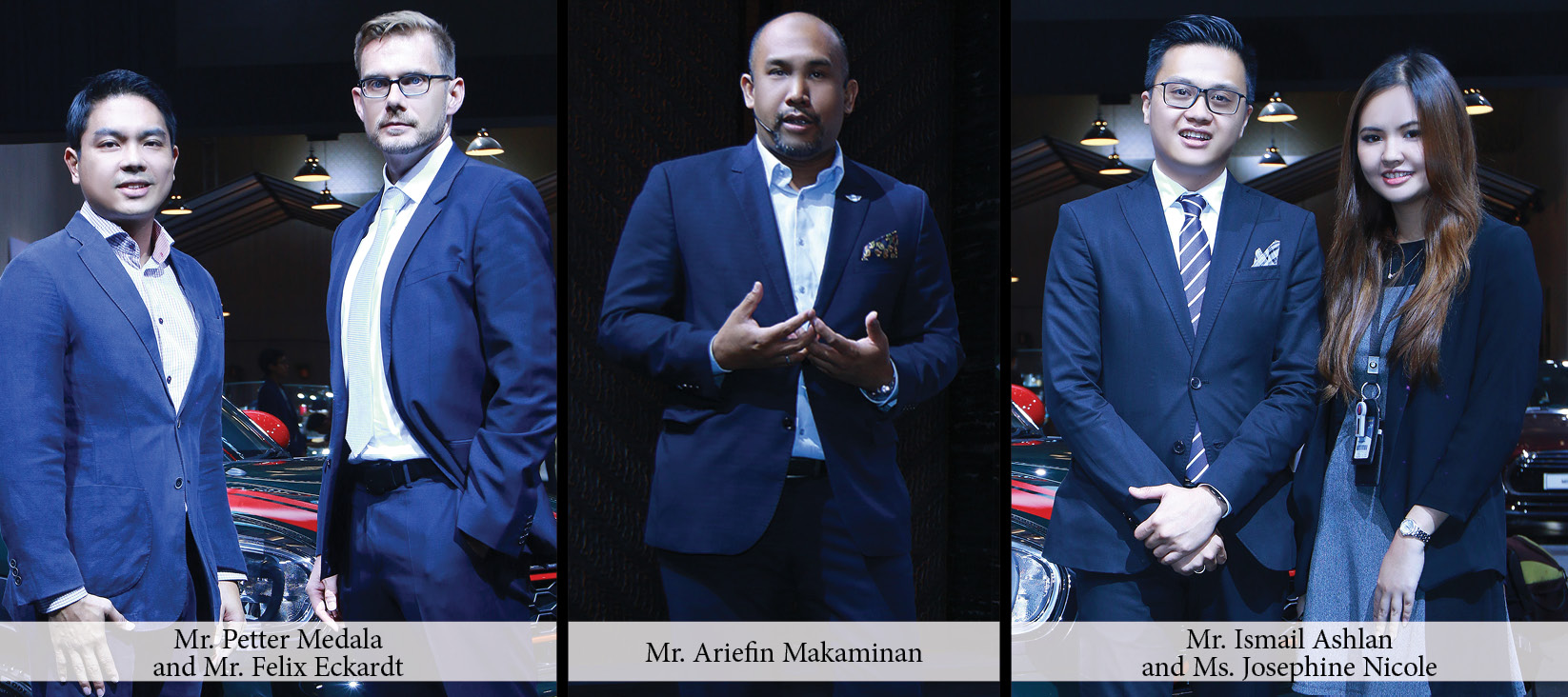The horizontal image is divided into three sections, each containing a professionally photographed image of individuals dressed in business attire, looking directly at the camera against dark backgrounds. The background includes reflections, suggesting the presence of a car with shiny red and blue metallic hues. 

The left section depicts Mr. Peter Medalla and Mr. Felix Eckhart. Mr. Medalla, who appears to be Asian with a short black cropped haircut, stands next to Mr. Eckhart, a tall white male with glasses and blonde hair. Both are wearing blue suits, and their names are displayed in a semi-transparent light gray rectangle caption at the bottom of the image.

The center section features a dark-skinned man with a bald head identified as Mr. Arifin Makaminian. He is wearing a dark blue suit with a white button-up shirt and a yellow handkerchief. His hands are interwoven in front of his chest, possibly mid-speech.

The right section shows Mr. Ismail Aichalan and Ms. Josephine Nicole. Both appear to be Asian, with Mr. Aichalan's hands clasped together in front of his body, and Ms. Nicole dressed in a suit with a dress underneath, standing neutrally. Their names are also displayed in a similar semi-transparent light gray rectangle caption at the bottom.

The overall composition, attire, and postures suggest this image might have been taken during a formal business conference or a photo opportunity.